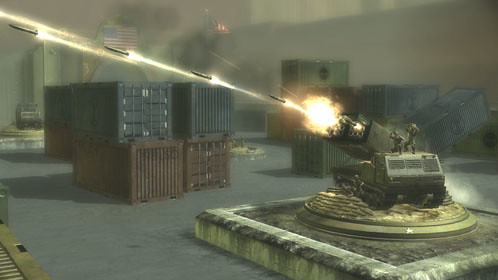This screenshot captures a dramatic moment in a cutting-edge 3D video game set in a gritty, industrial environment. Dominating the right side of the image, there is a massive automated turret, possibly mounted on a military vehicle, launching what appear to be large bullets or torpedoes. The backdrop includes an array of sizable shipping containers in blue and red, hinting at a utilitarian, metal-clad setting. The atmosphere is thick with smog or smoke, suggesting a heavily polluted area, likely a war zone. The image conveys a sense of intense action amidst a desolate and war-torn industrial landscape.